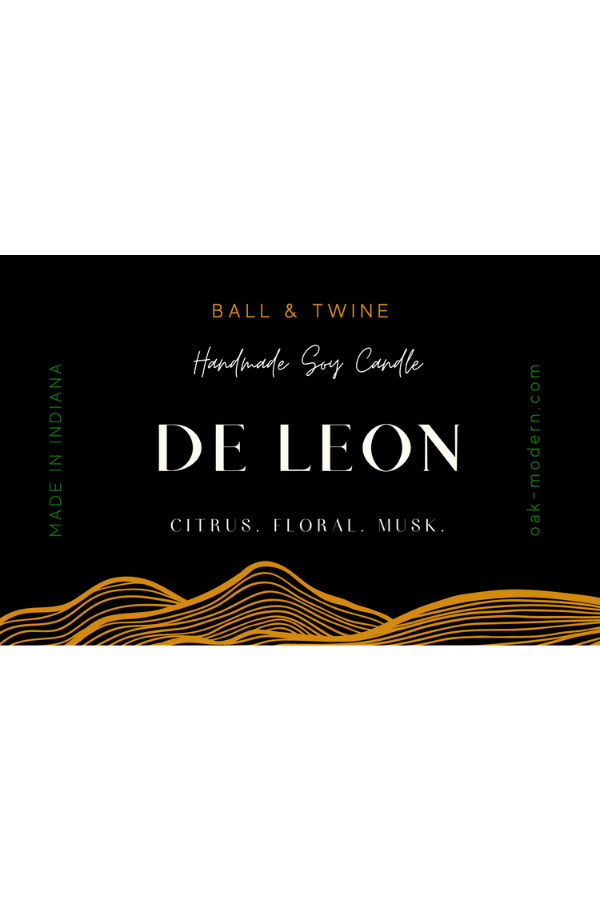The image is a sophisticated advertisement for a handmade soy candle. The background is solid black, creating a striking contrast with the white and orange text. At the top center, in bold orange font, it displays "Ball & Twine." Below this, in delicate white script, it reads "Handmade Soy Candle." Further down, in capitalized white letters, it states "De Leon." Beneath this, in smaller white font, are the words "Citrus · Floral · Musk." On the left-hand side, the phrase "Made in Indiana" is written vertically in green letters. Opposite, on the right-hand side, in the same green font, is the website address "oak-modern.com." The bottom fifth of the image features three orange wavy lines, reminiscent of waves or hills, adding a touch of visual interest to the otherwise minimalist design.